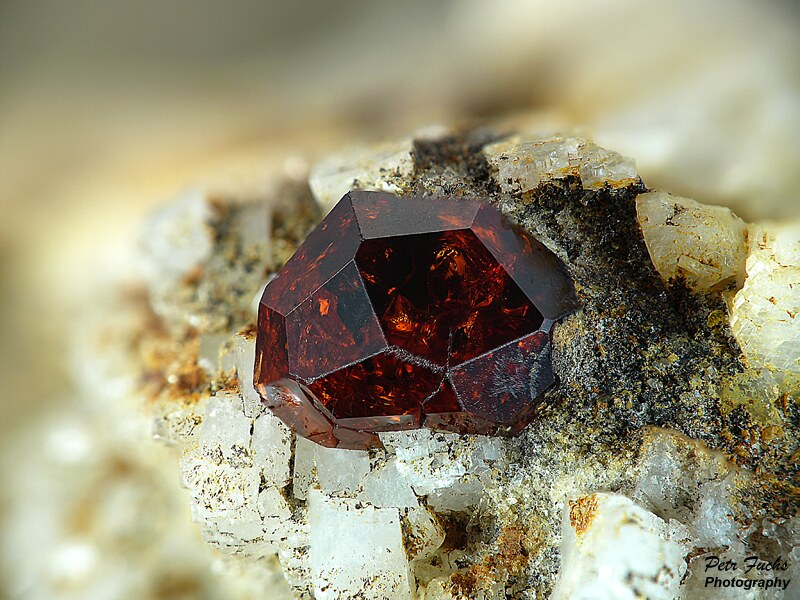The image depicts a striking gemstone emerging from a rough, rustic rock formation. The gem, a smooth, finely cut stone with octagonal facets, boasts vibrant hues of deep reds, oranges, and blacks, somewhat between ruby and garnet red. Its polished surfaces contrast sharply with the rugged textures of the surrounding rock, which is a blend of black, white, beige, and brown tones. The background is blurred, featuring a horseshoe-shaped pattern around the top, left, and bottom edges, with lighter grains and darker spots suggestive of sand or smaller crystals. A black text watermark reads "Pierre Tuck's Photography" in the bottom right corner.